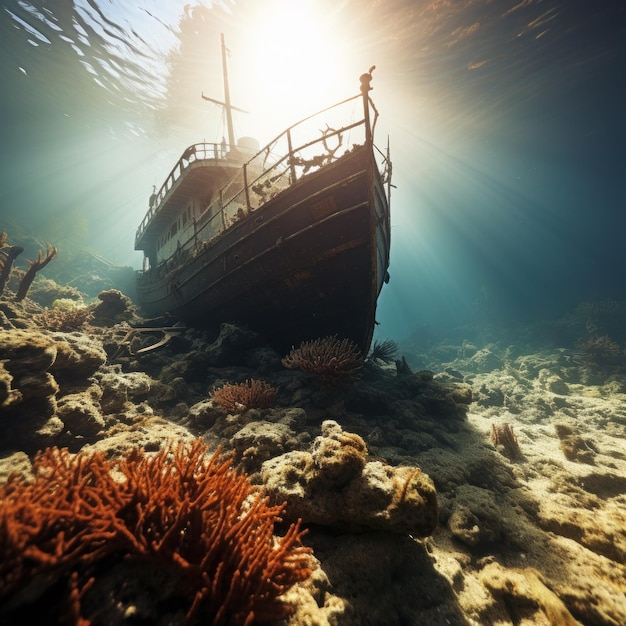An underwater vista captures the haunting image of a sunken ship resting on the ocean floor. Bathed in sunlight streaming through the rippling surface, it reveals a scene close to the water's top, indicating a relatively shallow depth. The ship, sizable and seemingly intact, boasts a dark hull—a mix of partly visible black and dark brown hues—contrasting with a white cabin structure above. A prominent mast, likely used for a radio, stands tall, equipped with metal railings now adorned with sparse coral and underwater microorganisms.

The foreground teems with vibrant marine life, including patches of red and white coral set against a sandy and rocky seabed. The ship's placement on the uneven terrain suggests a rough, rocky ocean floor. Despite the wear of time, the vessel shows minimal decay, indicating it hasn't been submerged long enough to suffer extensive deterioration. The overall scene, whether a realistic portrayal or an artist's rendering, projects both the charm and desolation of a ship caught between oceanic embrace and time’s relentless grasp.